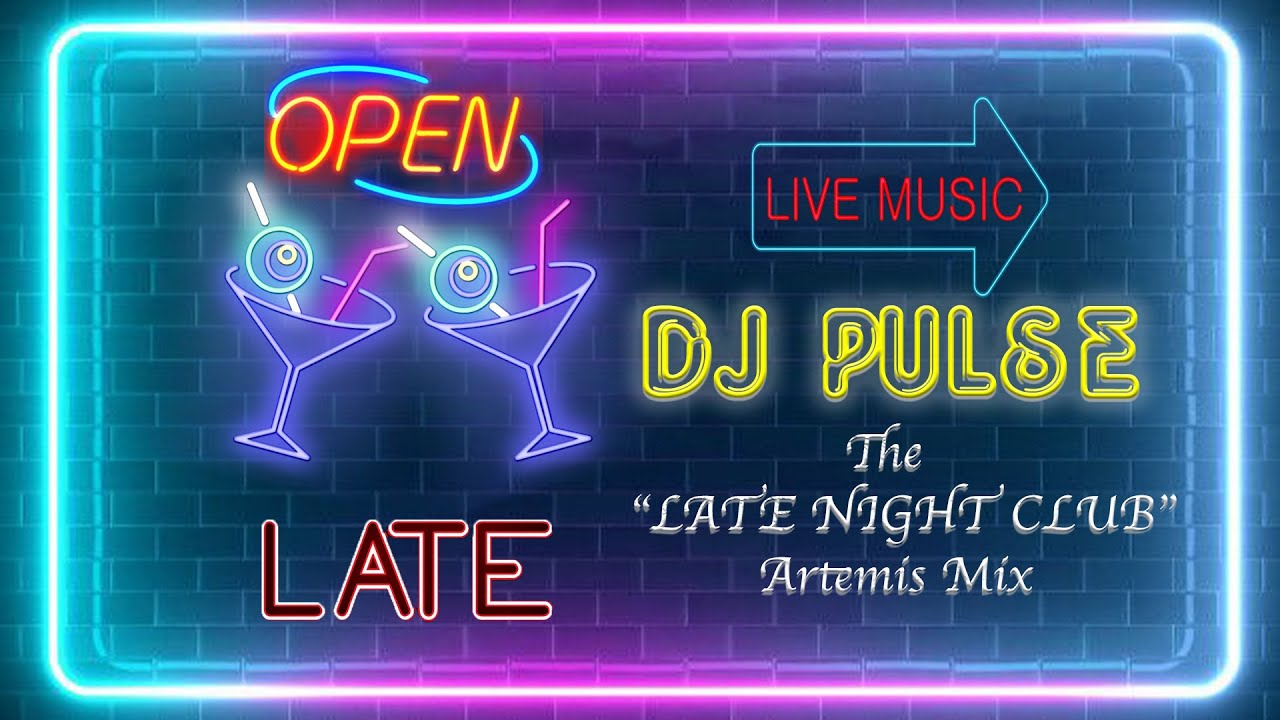This vibrant neon sign appears in the window of a bar or nightclub, featuring an array of eye-catching colors and details. Framed with turquoise, purple, and light blue neon lights, the sign prominently displays the word "OPEN" accompanied by two martinis with straws and olives. Beneath "OPEN," the word "LATE" is subtly included, though not illuminated. An arrow on the right side of the sign, in red lettering, announces "Live Music." Below the arrow, the name "DJ Pulse" is displayed in yellow neon, with the text "The Late Night Club" in white cursive, followed by "(Artemis Mix)" in parentheses. The sign's colorful scheme includes orange, purple, pink, blue, red, yellow, and white, making it stand out against a black and white brick background. The overall impression is that of a lively establishment open late, promising music and excitement.